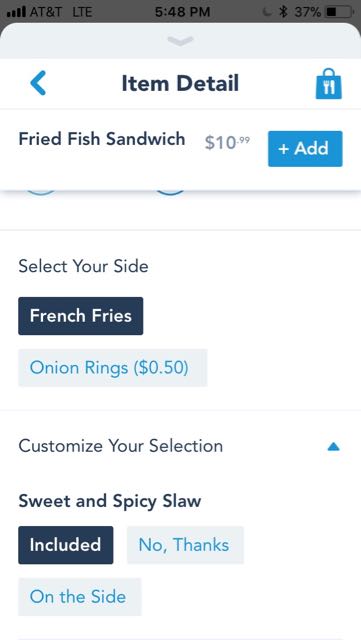A detailed, color portrait-format screenshot of a smartphone displaying a food ordering app at 5:40 a.m. The device, connected to AT&T with full signal bars, shows a battery life of 37%. The app is at the "Item Detail" section, featuring a menu with specific food options. Central to the screen is the listing of a Fried Fish Sandwich priced at $10.99, accompanied by an "Add" button to include it in the cart. Slightly lower on the screen is the "Select Your Side" section, currently showcasing French Fries. An option to add Onion Rings for an additional $0.50 is visible. The customization options for the order include Sweet and Spicy Slaw, which is currently included by default. The user can choose to remove it by selecting "No Thanks" or have it placed "On the Side." The overall app interface is predominantly white, with dark blue text for most of the writing. Interactive buttons, such as those for the French Fries and the customization options, feature a dark blue background with white text. The captured screenshot appears to have been taken after the user scrolled down to the latter part of the menu.